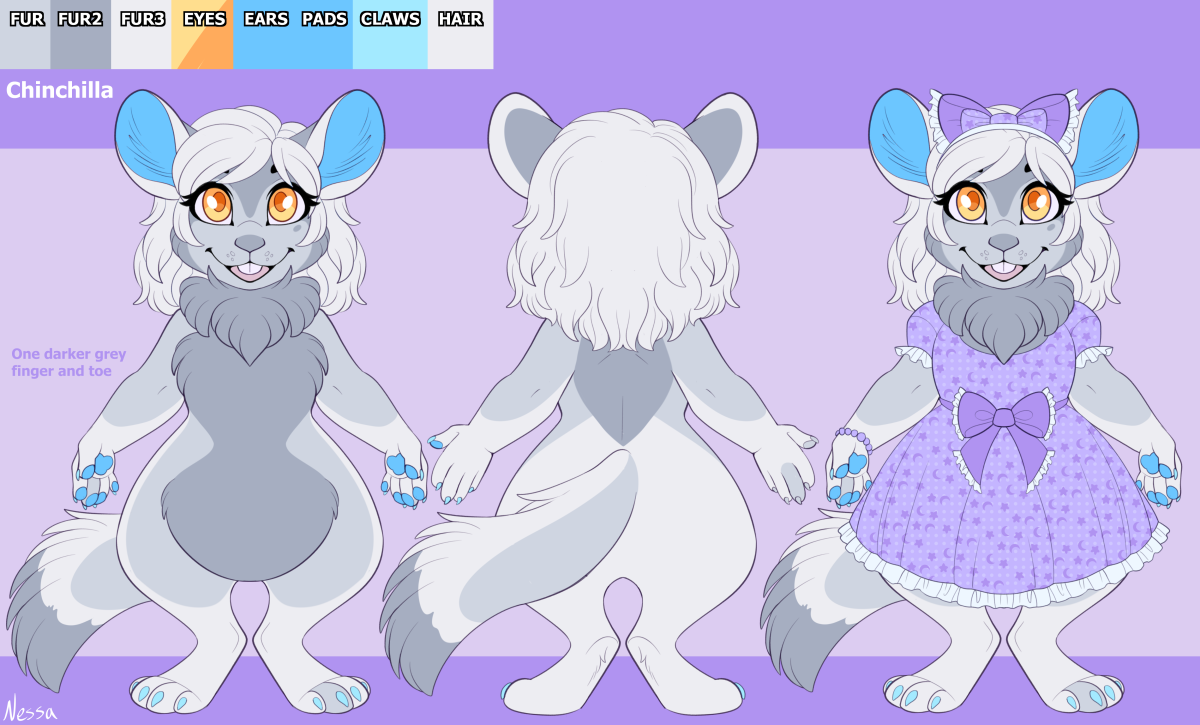The image is a detailed illustration of three cartoon chinchillas set against a two-tone purple background, where the top and bottom sections are dark purple, and the middle section is a lighter purple. The left side features white text that labels the image as "chinchillas." Each chinchilla is depicted with a combination of light gray, medium gray, and dark gray fur, featuring large, friendly brown eyes, and big ears. Their hands, feet, and claw pads are tipped with blue, and their toenails appear to be painted a lighter blue. 

The first chinchilla is facing forward, with a fluffy appearance around its neck but no clothing. The second chinchilla shows a back view, revealing a two-tone gray tail and mostly white back fur, with ears that are white and gray. The third chinchilla, also front-facing, is dressed in a purple dress adorned with a purple bow at the waist, and a matching bow with a small ball on top of her head.

Additionally, the image has a reference section at the top left, showing the colors used with labels such as fur, eyes, ears, pads, claws, and hair. The colors predominantly feature various shades of gray for the fur, orange for the eyes, blue for the ears and pads, lighter blue for the claws, and white or very light gray for the hair. Overall, the chinchillas are depicted as cute, friendly, and smiling characters.